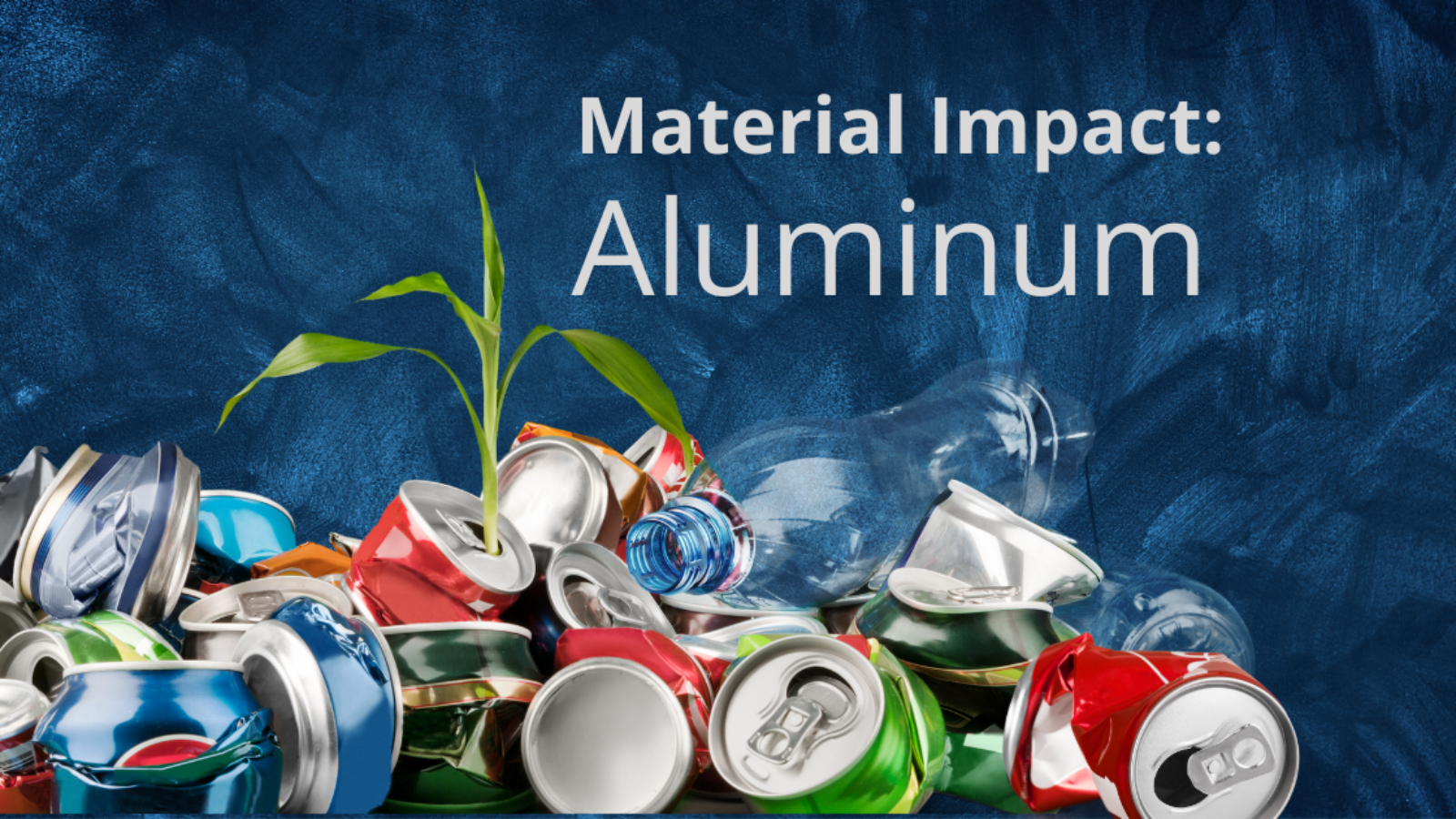The photograph captures an evocative scene centered on the theme of recycling, presented in a horizontal rectangular format. The background features an artistic blend of dark to medium blues, reminiscent of swirling paint strokes that harmonize to create a rich, textured backdrop. Prominently displayed in bold white lettering, the caption reads, "Material Impact: Aluminum."

In the foreground, a chaotic yet compelling pile of smashed soda cans dominates the scene. The cans, still bearing their tabs, are strewn haphazardly, emphasizing the magnitude of recyclables. Amidst this aluminum chaos, a single sprout of grass emerges with four distinct blades, symbolizing a glimmer of hope and renewal, sprouting from the remnants of consumer waste on the left side of the image.

Adding to the complexity, a plastic bottle can be spotted among the aluminum cans, subtly highlighting the inadvertent mixing of different recyclable materials. Another potential plastic bottle appears on the right, contributing an additional layer to the composition's narrative on waste and recycling.